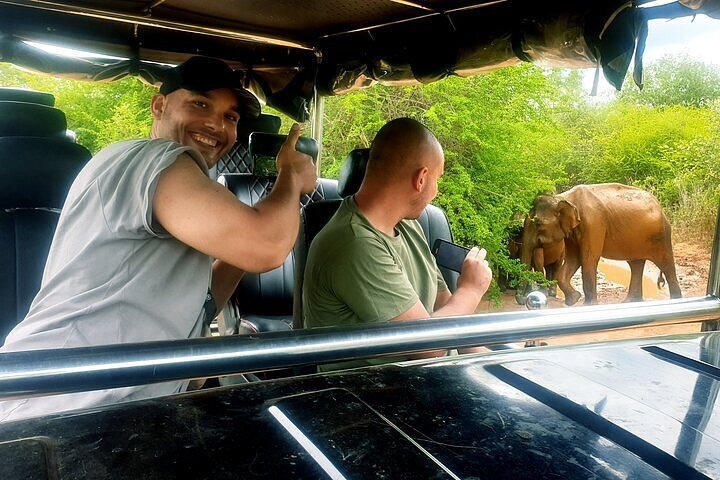The photograph features two men on a safari trip, sitting inside an open-roof, windowless truck with a fabric top, amidst lush green vegetation. The muddy brown path just outside the truck has a small patch of water, and nearby, there are two brown elephants, one of which is a baby, feeding in the brush. The man in the front passenger seat, dressed in a black cap and a white short-sleeved t-shirt, smiles at the camera with a thumbs up, not paying attention to the elephants. His companion, in the driver’s seat, wears a faded green short-sleeved t-shirt and is turned to his left, holding up a camera or phone, likely capturing a photo or video of the elephants. Both men appear engaged with their surroundings, capturing the moment.